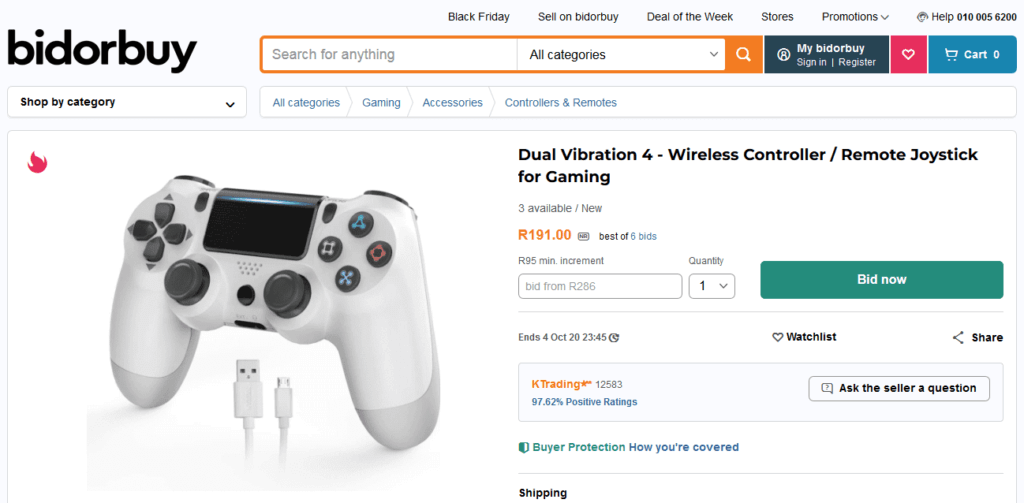Screenshot of an online auction listing on bidorbuy.com showcasing a wireless PlayStation Dual Vibration Controller/Joystick:

The primary image prominently displays a white PlayStation controller/joystick featuring gray buttons. The listing highlights that the item is new and currently available for bidding. The starting price is R191, with the highest bid at the moment recorded at R286. Bidders are required to place a minimum increment bid of R95. Potential buyers can place their bids through a green "Bid Now" button, and the auction ends on October 4th, 2020, at 23:45 (11:45 PM). 

Additional options include adding the item to a watchlist and sharing the listing. The seller, identified as K Trading, boasts a positive feedback rating of 97.82% based on 12,583 ratings. Buyer protection is offered for this purchase, and shipping details are available on the page. 

At the top of the webpage, users can find a search bar, highlighted with an orange box, allowing searches across all categories, including gaming accessories and controllers/remotes. A small fire icon in the corner of the listing image indicates that this is a hot sale item.